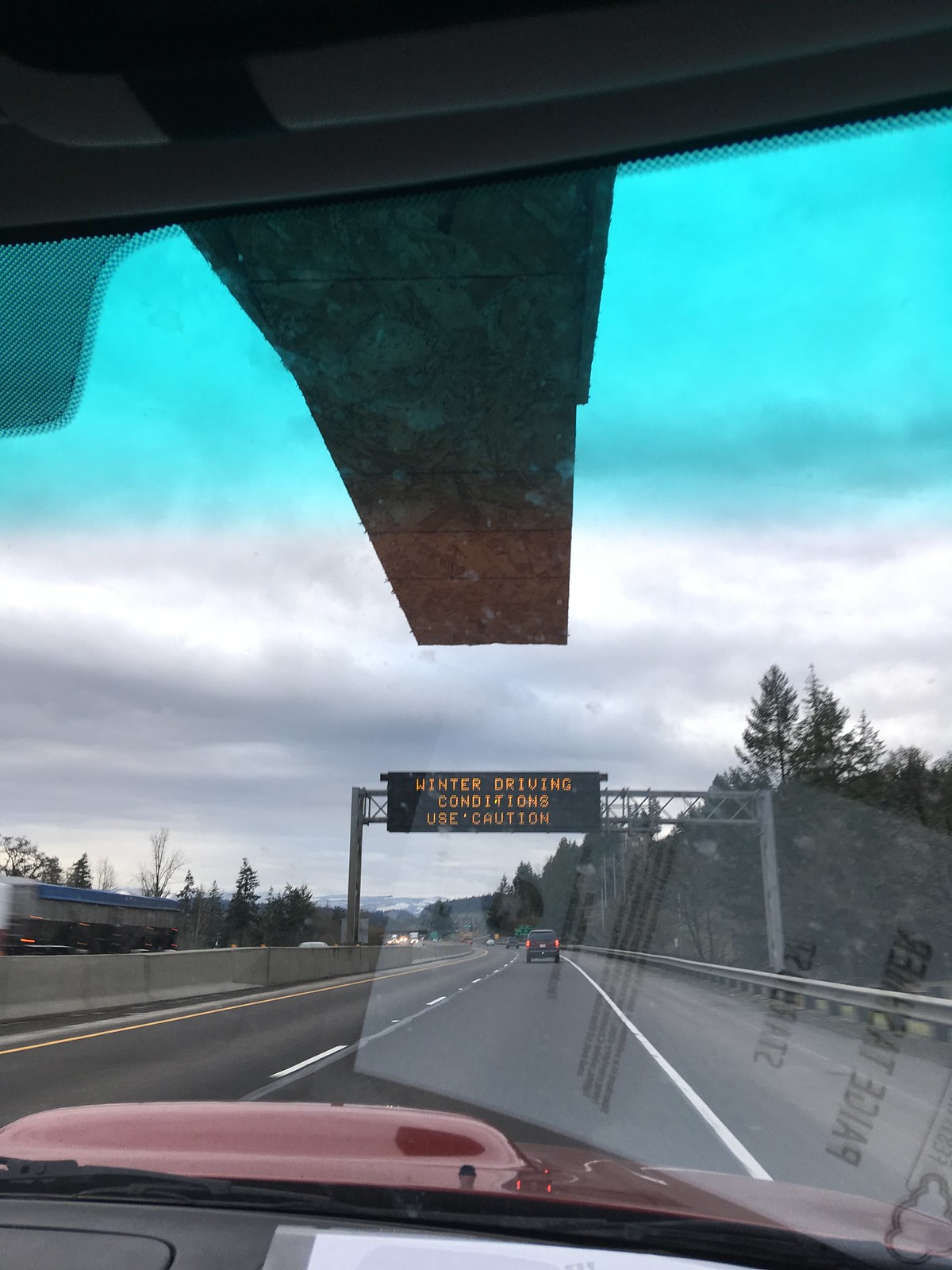The image appears to be taken from inside the passenger compartment of a vehicle, possibly a car or truck. Visible through the windshield is the vehicle's red hood, featuring a prominent central bulge likely designed to accommodate a larger engine. A reflection of a white sheet of paper with some indistinct black writing can be seen on the windshield, positioned above a dark-colored dashboard.

The vehicle is driving on an asphalt roadway marked by a solid white line on the right and a dashed white line in the center, delineating two lanes of traffic. To the left, a concrete partition separates oncoming traffic. Oncoming vehicles, including some with visible headlights, can be seen beyond the partition.

An illuminated black road sign is mounted on two posts that extend across the roadway. The sign displays a warning in yellow letters: "Winter Driving Conditions Use Caution." The sky is overcast, indicating a cloudy day, and the overall ambiance suggests daytime despite the heavy cloud cover.